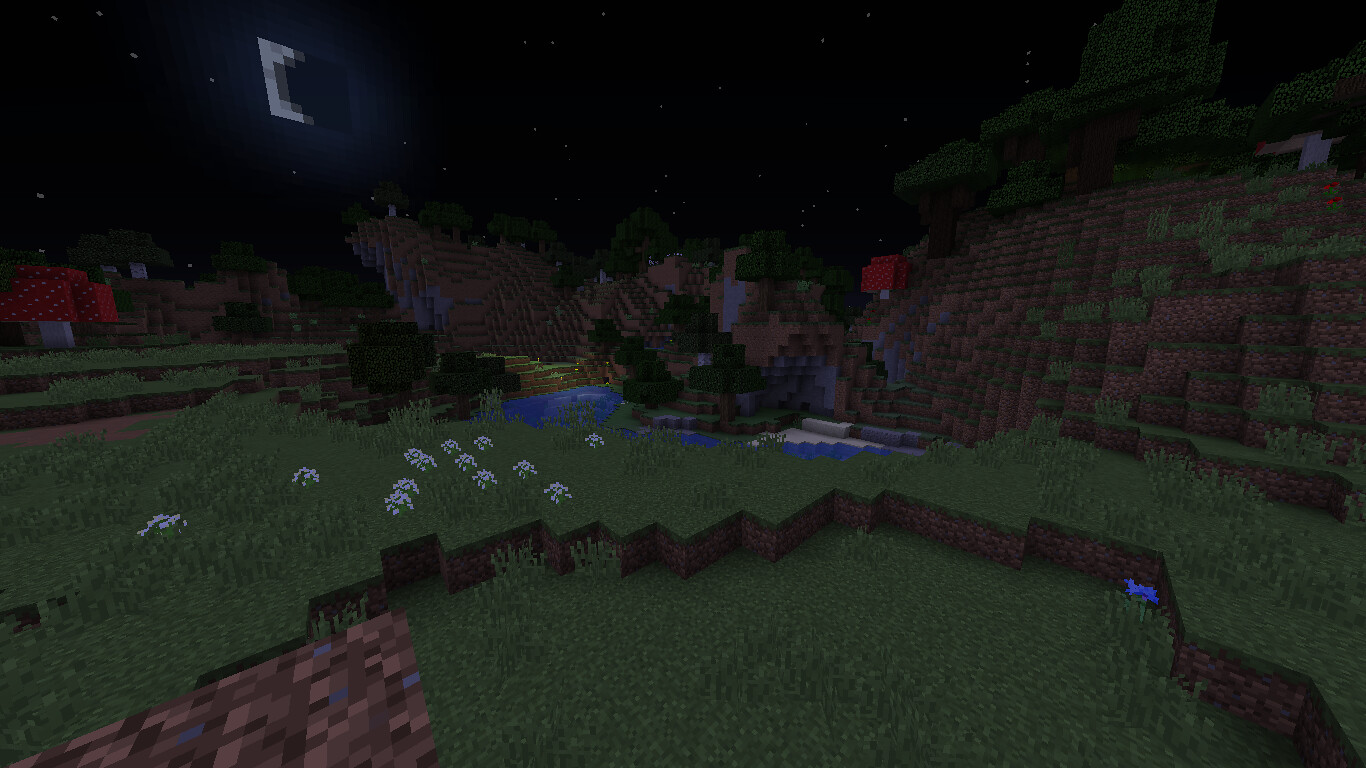The image appears to be a screenshot from a gaming device, though it is somewhat blurry. In the bottom left corner, there is a small, hand-drawn brick wall that transitions into a patch of dark green grass. This grassy area is bordered by a dark brown wall, with some sections of the grass appearing longer than others. Scattered across the grassy field are tiny white dots, potentially indicating animals or small objects.

In the background, a mountainous landscape is visible. The mountain is predominantly brown with patches of green, suggesting vegetation, and streaks of red, dark brown, and black are also interspersed across it. To the left of the mountain, there seem to be brown and red structures that could be buildings. The entire scene is set against a black sky dotted with tiny white specks, likely representing stars.

There is also a peculiar half-box or C-shaped element at the top left corner of the image, which is brightly lit in white, although its purpose or identity is unclear. The scene conveys a sense of a quiet, possibly rural setting under a starry night sky, complete with grassy fields, distant mountains, and a few scattered buildings.